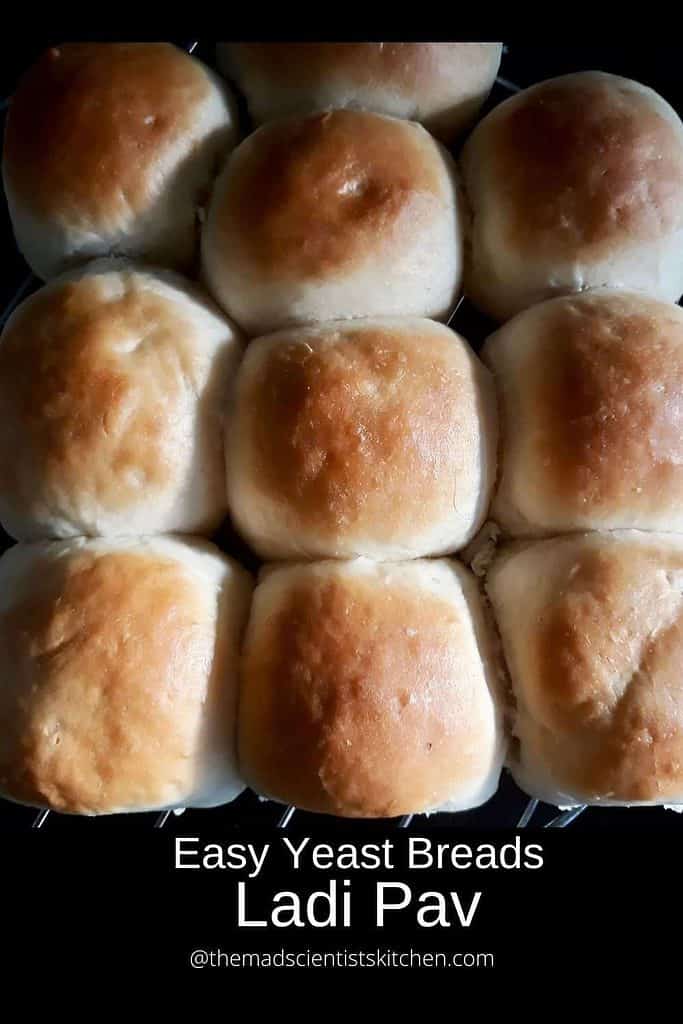The image features a collection of ten freshly baked Ladi Pav yeast rolls, arranged with one roll at the top, followed by three rows of three. Each roll boasts a beautifully toasted, brownish-orange top, giving way to creamy-colored sides. The tops of some rolls display a shiny finish, indicating they might have been brushed with butter or an egg wash before baking. The rolled breads rest on a wire rack, evident from the steel wires visible in the image. Across a black background at the bottom, the text reads: "Easy Yeast Breads, Ladi Pav," followed by "at TheMadScientistKitchen.com."